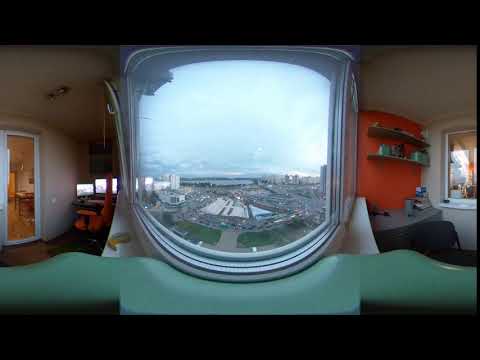The image is a rectangular indoor photograph capturing a room with patio doors and windows on the left side, alongside a white wall and a glass door leading outside. On the right side is an orange wall with floating dark brown shelves holding various items. Below the shelves is a table with some books, adjacent to another window. In the center of the room is a striking mirror that creates the illusion of a circular window, revealing a panoramic cityscape. This cityscape includes a large array of buildings, roadways, green spaces, and water, beneath a partly cloudy, grayish-blue sky. The vivid reflection juxtaposes the indoor setting with the outdoor urban vista, blending the domestic space with the distant skyline, thereby creating a sense of depth and contrast within the photograph.